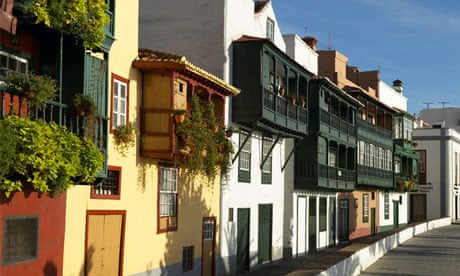The image captures a picturesque European street lined with quaint, closely situated homes. Predominantly featuring shades of red, yellow, white, and tan, these buildings sport a mix of hunter green trimmings and accents. The white houses, some reaching up to three stories high with attics, are particularly eye-catching with their neatly structured balconies, adorned with hanging greenery. The balconies, which are mostly black or hunter green, are found primarily on the second or third stories, with some buildings boasting dual levels of balconies. The street follows a gentle curve, creating a charming, uninterrupted view down its length. 

An elevated sidewalk runs parallel to the street, providing a distinct separation from the road. The vibrant blue sky and bright sunlight suggest a pleasant spring or summer day. The rooftops, adorned with antennas, add to the authentic European feel of the scene. Noticeably, there are no storefronts or commercial signs visible, reinforcing the residential vibe of the area. The overall composition of the image, with its detailed architectural features and verdant touches, offers a serene glimpse into daily life in a picturesque European neighborhood.